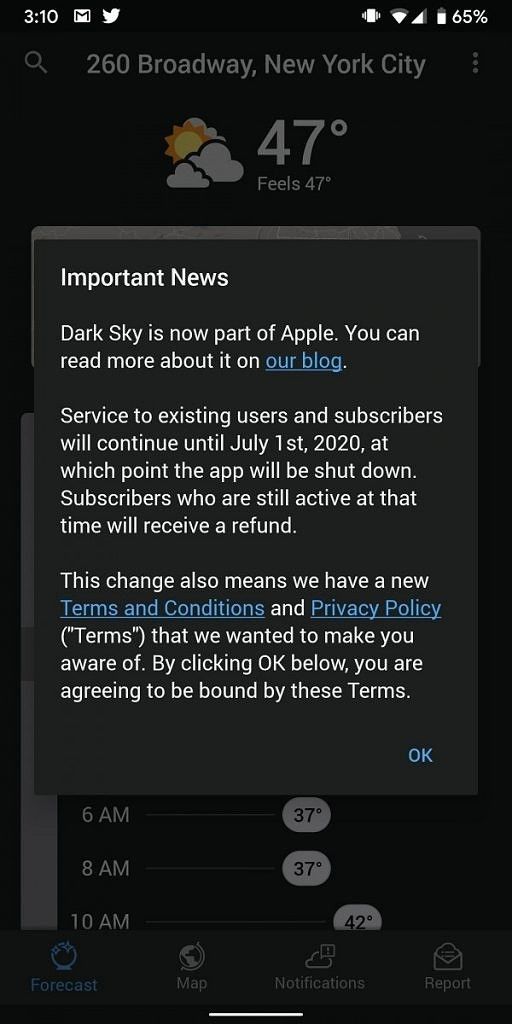The image is a vertical screenshot taken on a mobile phone. The status bar at the top exhibits the time as 3:10, with a battery charge of 65%. The background is a dark gray hue.

At the top of the image, the location "260 Broadway, New York City" is displayed, along with the current weather information: 47 degrees, feels like 47 degrees. An icon depicts the sun partially obscured by two clouds, with an additional cloud in the background.

Below this, a dark gray rectangle with white text conveys an important announcement: "Dark Sky is now part of Apple. You can read more about it on our blog. Service to existing users and subscribers will continue until July 1st, 2020, at which point the app will be shut down. Subscribers who are still active at that time will receive a refund. This change also means we have a new Terms and Conditions and Privacy Policy (Terms) that we wanted to make you aware of. By clicking OK below, you are agreeing to be bound by these terms." An "OK" button is present for users to acknowledge this message.

Further down, a row of time-specific temperatures is detailed: 6 a.m. at 37 degrees, 8 a.m. at 37 degrees, and 10 a.m. at 42 degrees.

At the bottom of the screenshot, a dark gray strip features four icons with accompanying text, reading from left to right: "Forecast," "Map," "Notifications," and "Reports."